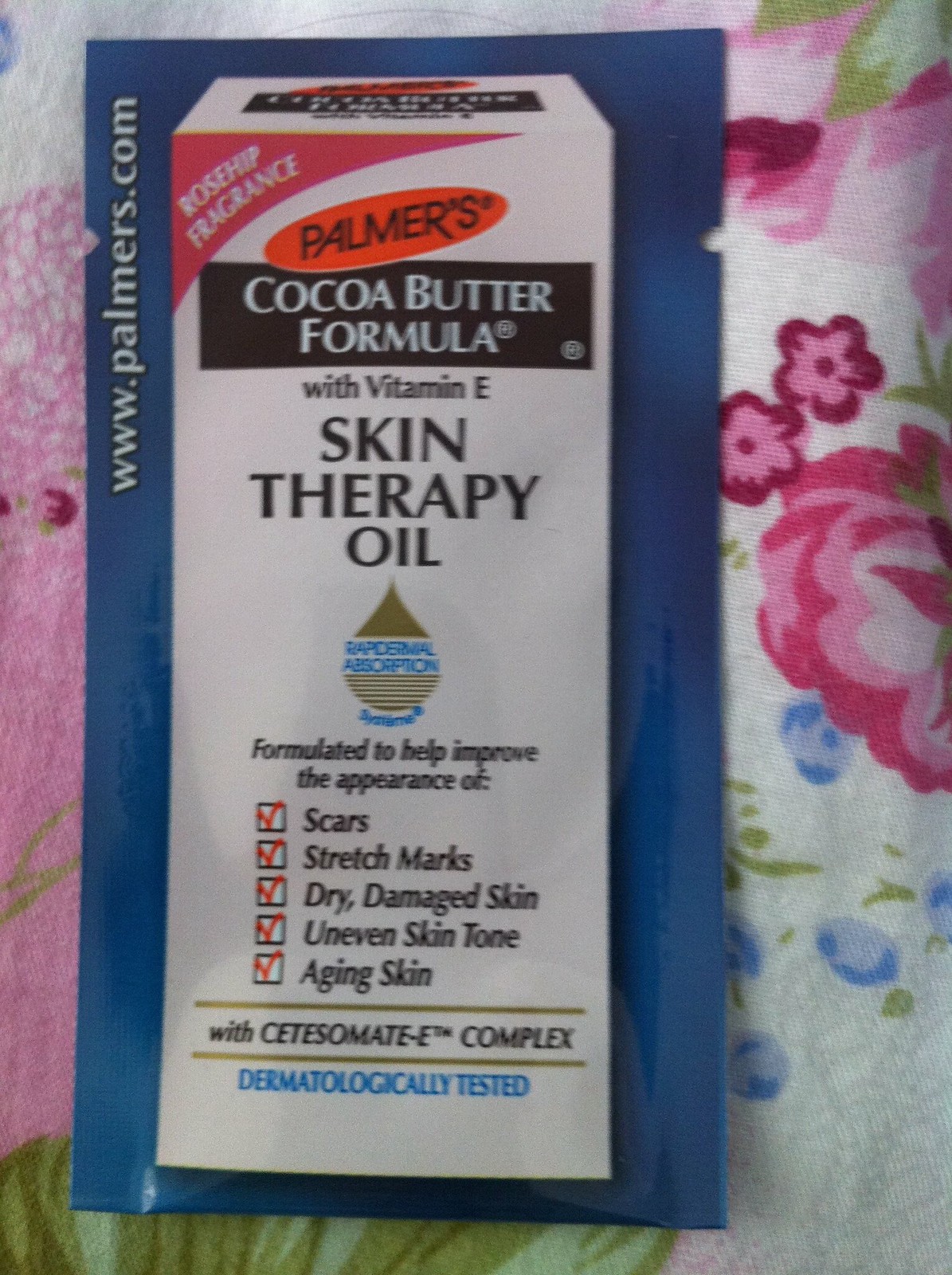The image depicts a colorful, vertical rectangular package of Palmer's Skin Therapy Oil. The product is encased in clear plastic with a blue backing and features a predominantly white label. At the top left corner, the web address "www.palmers.com" is visible, along with the mention of a Rosehip Fragrance. Central to the design is an orange circle with the Palmer’s logo, followed by a black rectangle containing white text that reads "Cocoa Butter Formula." Beneath that, in brown text, it states "With Vitamin E" and "Skin Therapy Oil." The lower part of the label details the product's benefits, stating it helps improve the appearance of scars, stretch marks, dry and damaged skin, uneven skin tone, and aging skin. These benefits are listed with checked boxes in orange. Additionally, it highlights that the oil is formulated with the Cetasomate-E Complex and is dermatologically tested. The package is photographed against a bright, flowery fabric, making the image clear and vibrant.